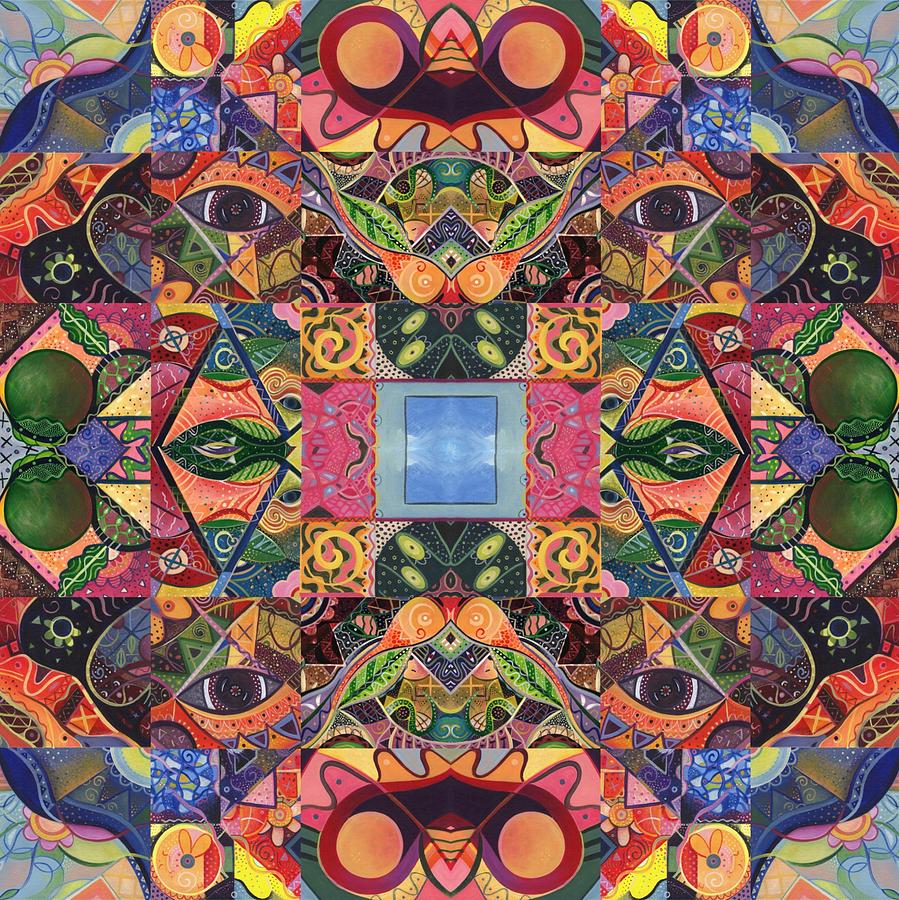The image depicts a vibrant and intricate artwork divided into numerous multicolored squares, each hosting a variety of colors such as red, blue, green, orange, and peach. At the center lies a prominent sky-blue square, surrounded by a nearly rectangular pink square filled with varied objects and patterns. The overall composition resembles a kaleidoscope, showcasing symmetrical and harmonious designs that repeat across the image. Notably, the far right square contains two green spherical objects, which reappear at the top and bottom of the artwork in a peach-like hue. Additionally, a recurring eye pattern is visible in each of the four corners. The artwork features complex abstract designs, including yellow swirls, purple eyes, green leaves, and a pomegranate leaf motif, all contributing to its rich and colorful aesthetic. The entire piece exudes a sense of creative synthesis, blending colors and patterns in a visually engaging manner reminiscent of both kaleidoscopic imagery and magic eye illusions.